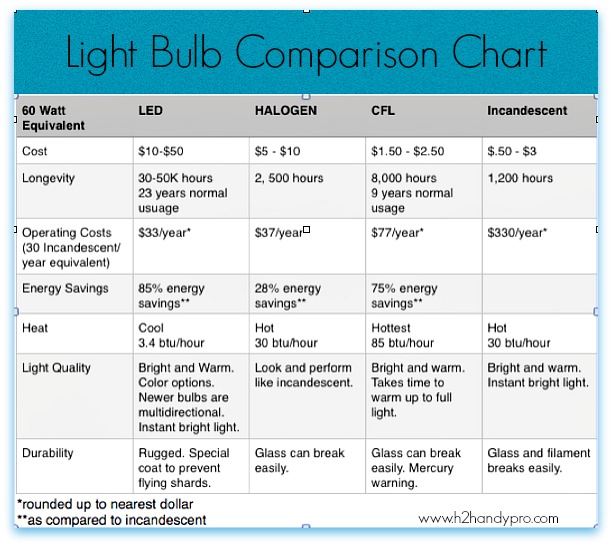This detailed light bulb comparison chart, designed as an informational poster, features a blue header with the title "Light Bulb Comparison Chart" in black text. The chart itself is organized in gray and white backgrounds with black font for clarity. It is divided into five primary columns under a gray sub-header listing: "60 Watt Equivalent," "LED," "Halogen," "CFL," and "Incandescent." Each column compares several attributes of these lightbulb types, including cost, longevity, operating costs, energy savings, heat generation, light quality, and durability. For example, the cost comparison shows LED bulbs at $10-$50, halogen bulbs at $5-$10, CFL bulbs at $1.50-$2.50, and incandescent bulbs at $0.50-$3. The chart includes additional benchmark comparisons such as "30 incandescent year equivalent" and provides detailed analysis through rows. At the bottom, there are footnotes marked with asterisks indicating rounded costs and comparisons to incandescent bulbs. The chart concludes with the website www.h2handypro.com, suggesting it could be a resourceful tool for both DIY enthusiasts and professionals in selecting appropriate lighting solutions for various uses around the home or office.